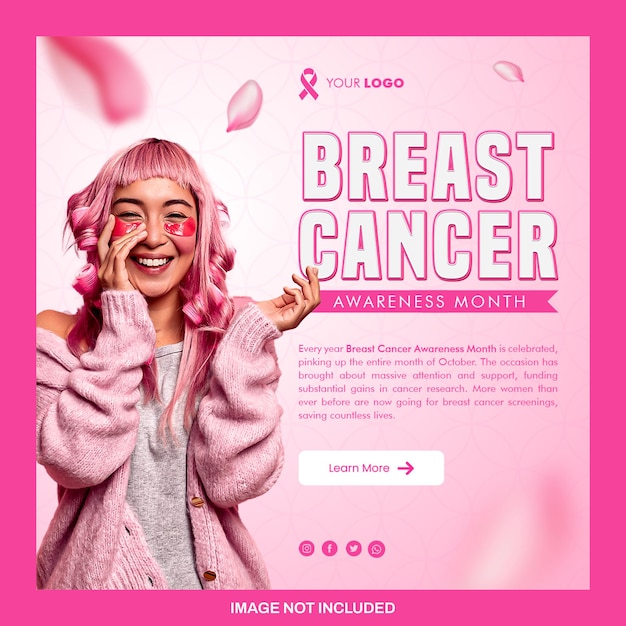The image features a vibrant Barbie pink border, framing the content within. On the left side, a young woman is pictured wearing a pink sweater, matching pink hair rollers, and pink under-eye masks designed to reduce puffiness. Her hair is also dyed pink, embracing the theme thoroughly. 

To her right, large bold letters declare "Breast Cancer Awareness Month." Beneath this, smaller pink text explains the imminent arrival of Breast Cancer Awareness Month and invites viewers to sponsor, contribute, or donate to breast cancer research. The information emphasizes the opportunity for potential sponsors to support the cause by featuring their logo next to the prominent pink awareness ribbon displayed at the top of the image. A white clickable button is also present, providing a call-to-action for more information about sponsorship opportunities. The design serves as an outreach initiative to garner support and raise awareness for Breast Cancer Awareness Month.